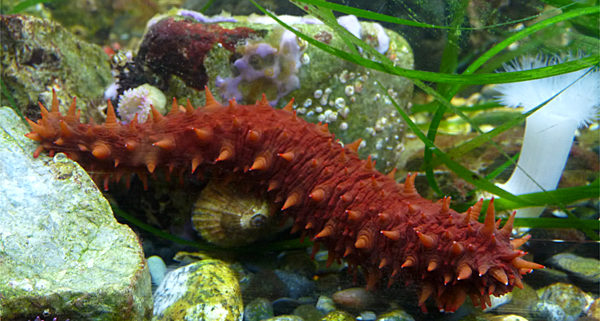The image showcases a vividly clear underwater scene, characterized by a serene marine environment. The bottom is dotted with smooth pebbles and adorned with delicate, white aquatic plants. Interspersed among them are strands of green, grass-like vegetation, adding to the lush underwater landscape. At the heart of the image lies the focal point: a striking, elongated sea slug-like creature. This red, worm-like entity is almost entirely covered in a myriad of sharp spikes, giving it a formidable appearance. However, a portion of its back is noticeably smoother. The creature's impressive length is accentuated by its proximity to several visible shells, which appear diminutive in comparison. Positioned with an orientation seemingly directed to the right, the creature presents an enigmatic profile, lacking discernible facial features.